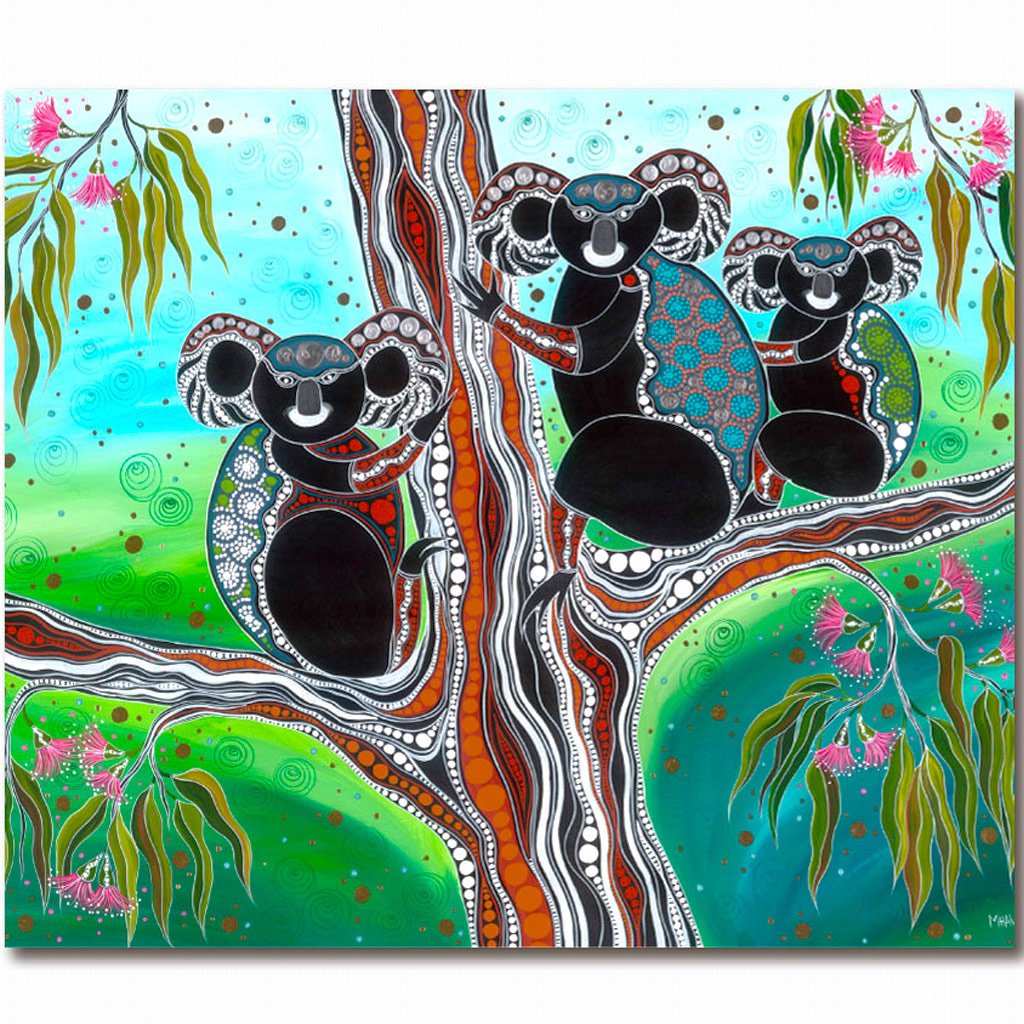The artwork is a vibrant, psychedelic depiction of three koala bears resting on a tree, rendered in a modern, abstract style. Dominated by an explosion of colors, the background is filled with shades of green signifying lush foliage, blues representing the sky, and pink buds highlighting the presence of flowers. The tree trunk and branches are illustrated with wavy lines and intricate geometric patterns in hues of brown, red, and black, giving it a surreal, almost hallucinatory texture. Dot-like particles in brown are scattered across the background, enhancing the forest-like atmosphere. 

The koalas themselves are a striking focal point, painted in a myriad of colors. Their faces and ears are adorned with jewel-like patterns in black and silver, and their heads feature diamond designs. The bodies of the koalas exhibit a mosaic of colors: teal, green, red, and black, blending into geometric and turtle shell patterns on their limbs and bellies. The detailed rendering extends to their forearms and calves, which showcase red and white patterns. Despite the abstract, fanciful style, the essence of the koalas is unmistakable, capturing their distinct characteristics amid the artistic chaos. 

A barely discernible signature occupies the bottom right corner of the piece, adding a personal touch from the artist. The artwork is presented against a white wall, emphasizing its vivid, dynamic nature.